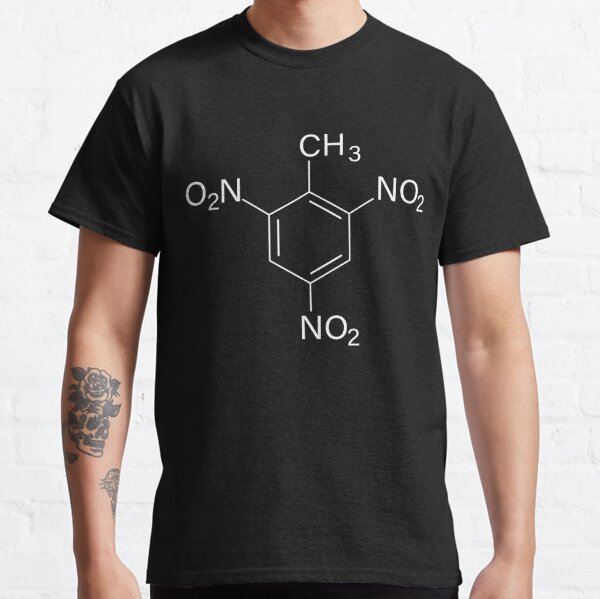The image is an advertisement for a black t-shirt adorned with a white scientific design on the front. The design features a six-sided molecular structure with chemical notations including O2NCH3NO2 and NO2, suggesting it represents a complex chemical compound. The model wearing the t-shirt has light skin and a distinctive tattoo on their right arm, depicting a skull with a flower emerging from it. The model’s face and lower half are not visible, focusing attention on the t-shirt itself. The background is off-white, providing a neutral backdrop that emphasizes the shirt. This minimalistic, professional image appears to be intended for an online retail store selling this scientific-themed t-shirt.